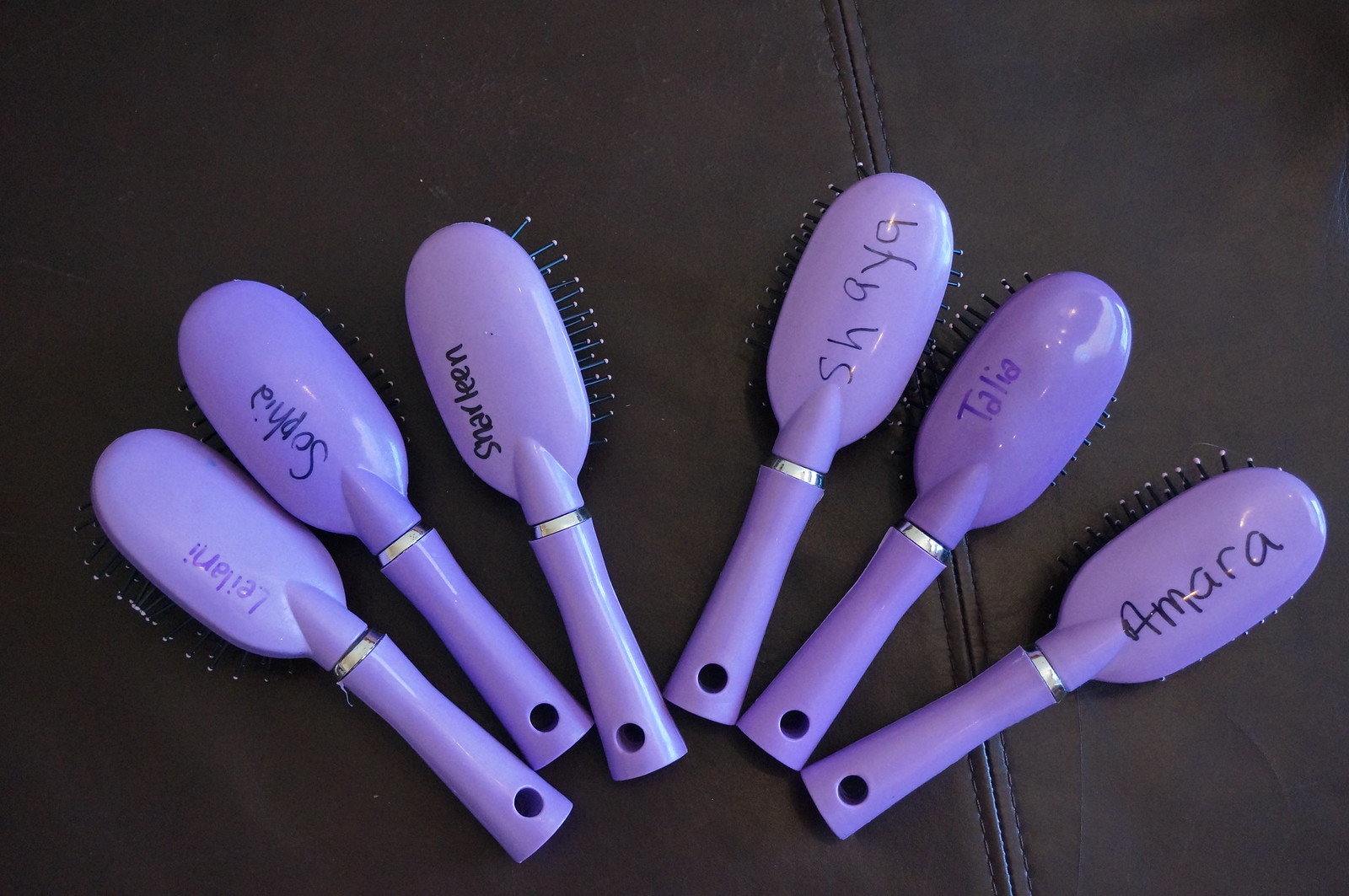This is a detailed photograph of six identical, light purple plastic hairbrushes with black bristles, displayed face down on a dark brown to black leather or faux-leather surface. Each brush features a small silver band between the handle and the brush head, as well as a hole at the very base of the handle. The bristles, though mostly obscured, have lavender tips and small balls at the ends. The brushes are laid out in a slight arc, creating a fan-like arrangement with handles pointing towards the bottom center of the image. The brushes are meticulously labeled with names: from left to right, the first is marked “Leilani” in purple marker, followed by “Sophia” in black, “Charlene” also in black, “Shaya” in black, “Talia” in purple, and finally “Amara” in black. They rest on a leather surface featuring visible stitching and seams, adding to the composition's texture and detail.